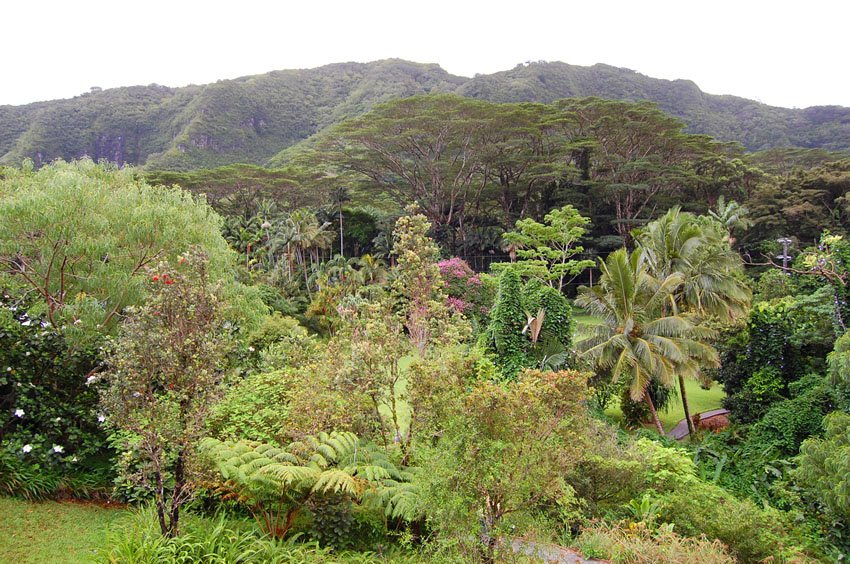This photograph captures an elevated view of a luxuriant, densely forested tropical area, possibly reminiscent of Hawaii or Puerto Rico. The image showcases a harmonious blend of light and dark green vegetation, creating a rich canvas of tropical foliage. In the foreground, palm trees gracefully rise above a variety of tropical plants, including low, palm-like shrubs and Mandevilla-type flowering shrubs displaying their red and white blossoms. Nestled to the left, a well-maintained yard, adorned with a pathway and possibly lit by a distant power pole or a lamppost, adds a human touch to this natural setting.

As the scene extends downward, the greenery intensifies, comprising flowering bushes with pink and purple blooms. These lush plants converge into a verdant valley, surrounded by taller trees whose canopies create a flat, fan-like appearance, fostering an impression of a living roof over the lower flora. The tropical foliage extends to the backdrop where a steeply sloped, rounded mountain appears, draped in thick rainforest vegetation. Further beyond, another upward-sloping mountain forms the horizon line, its tree-laden slopes yielding to a sky that transitions from a very light blue to nearly white where it meets the mountain peaks. The entire composition radiates a serene, vibrant energy, an emblem of tropical paradise.